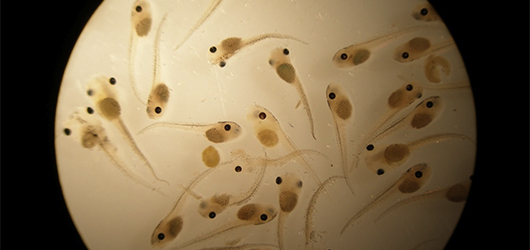The image, viewed under a microscope, showcases a rectangular frame with pure black borders on the left and right sides. Dominating the center is a smooth, tan-colored circular section. Inside this section, there are about 15 tadpole-like creatures, each with long tails and two prominent black eyes. The creatures vary in shades from off-white to dirty yellow to dark brown. Arranged in various directions—north, south, east, and west—they appear to be swimming around within the tan circle. Their semi-transparent bodies reveal a darker tan center, creating a vivid contrast against the background.